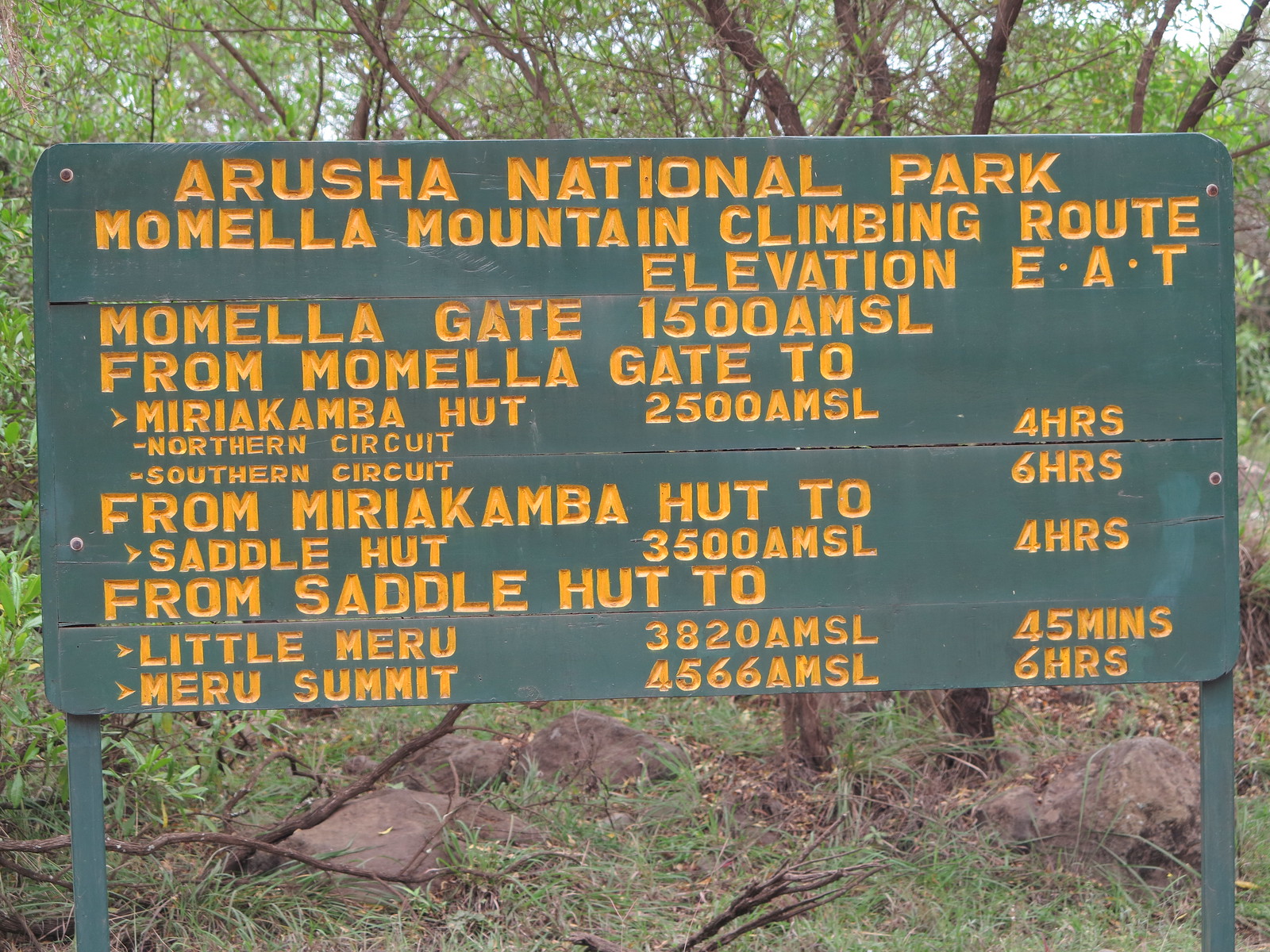The image depicts a wooden sign located in a wooded, grassy area, suggesting an entrance to a National Park. The sign is painted light green with dark green support legs on each side, and prominent yellow lettering at the top. It reads "Arusha National Park, Momella Mountain Climbing Route." Various elevation points and hiking details follow: "Momella Gate, 1500 AMSL; from Momella Gate to Mirakamba Hut, 2500 AMSL - Northern Circuit, 4 hours, Southern Circuit, 6 hours; from Mirakamba Hut to Saddle Hut, 3500 AMSL, 4 hours; from Saddle Hut to Little Meru, 3820 AMSL, 45 minutes; and Meru Summit, 4566 AMSL, 6 hours." The background consists of trees, indicating a natural, forested environment.